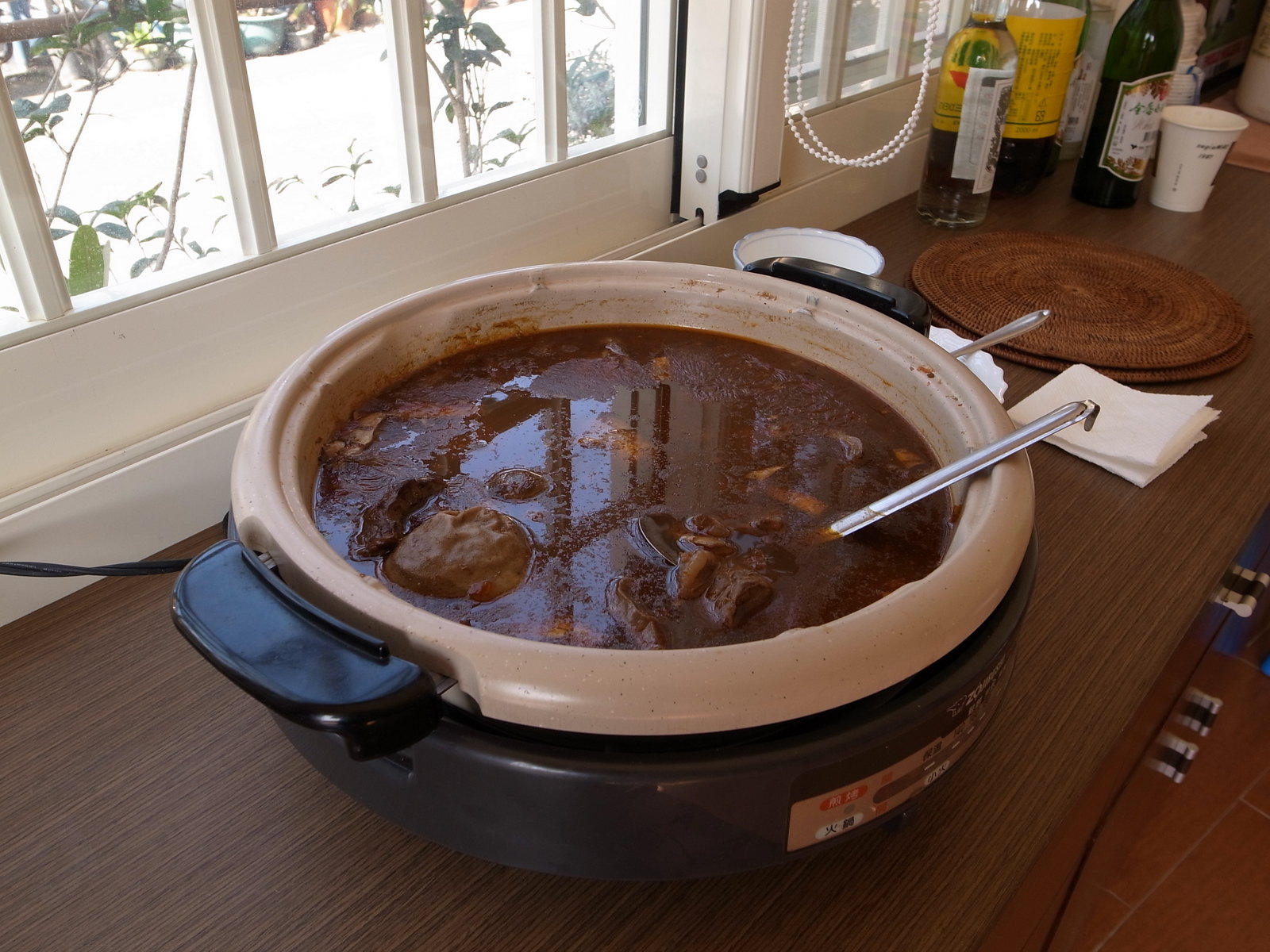The image showcases a homely indoor setting, with a view through bright white windows with white casing, almost washing out the outside scene. In the foreground, sitting on a brown, wood grain countertop, is a blue pot with black handles—one handle faces the left corner and the other points towards the upper right. Inside the blue pot is another white pot containing a hearty, brown beef stew, rich with chunky ingredients like meat or potatoes. A metal spoon hangs out from the pot. Beyond the pot, to the left, there is a green wine bottle with a white label, a yellow bottle, and a white paper cup. The reddish-orange tiled floor is also visible. Through the small-paned window in the background, leaves can be seen, adding a touch of greenery to the otherwise indoor scene.